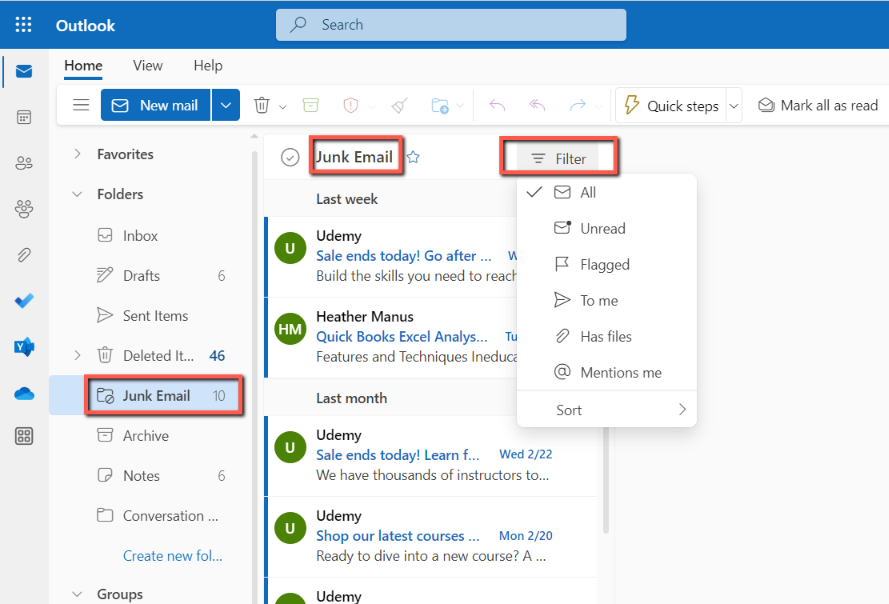In this image, we see a detailed view of an individual's Outlook email interface. At the top, there's a blue banner displaying "Outlook" along with a search icon. Directly below the banner are menu choices labeled Home, View, and Help. The main section of the interface focuses on composing a New Mail.

On the far left, there is a sidebar with various icons providing navigation to different parts of Outlook, such as mail, contacts, and attachments. Further down this sidebar, there is a menu featuring Favorites and Folders.

Within the Folders section, several categories are listed:
- Inbox
- Drafts (containing 6 items)
- Sent Items
- Deleted Items
- Junk Email, which is highlighted with a red border and indicates 10 unread messages
- Archive
- Notes
- Conversation History
- Create New Folder

There is also a Groups category.

Currently, the view is set to display the Junk Email folder, filtered to show All items. Four specific emails are visible in this folder:
1. An email from Udemy titled, "Salence Today: Go After, Build the Skills You Need to Reach."
2. An email from Heather Manners concerning "QuickBooks: Excel Analysis or Analyst, Features and Techniques in Education."
3. Another email from Udemy from last month with the subject, "Salence Today: Wednesday, 2-22, We have thousands of instructors to..."
4. A third email from Udemy dated Monday, 2-20 titled, "Shop Our Latest Courses: Are You Ready to Dive Into a New Course?"

The image presents a comprehensive look at the user's organizational structure within Outlook and highlights specific details within the Junk Email folder.